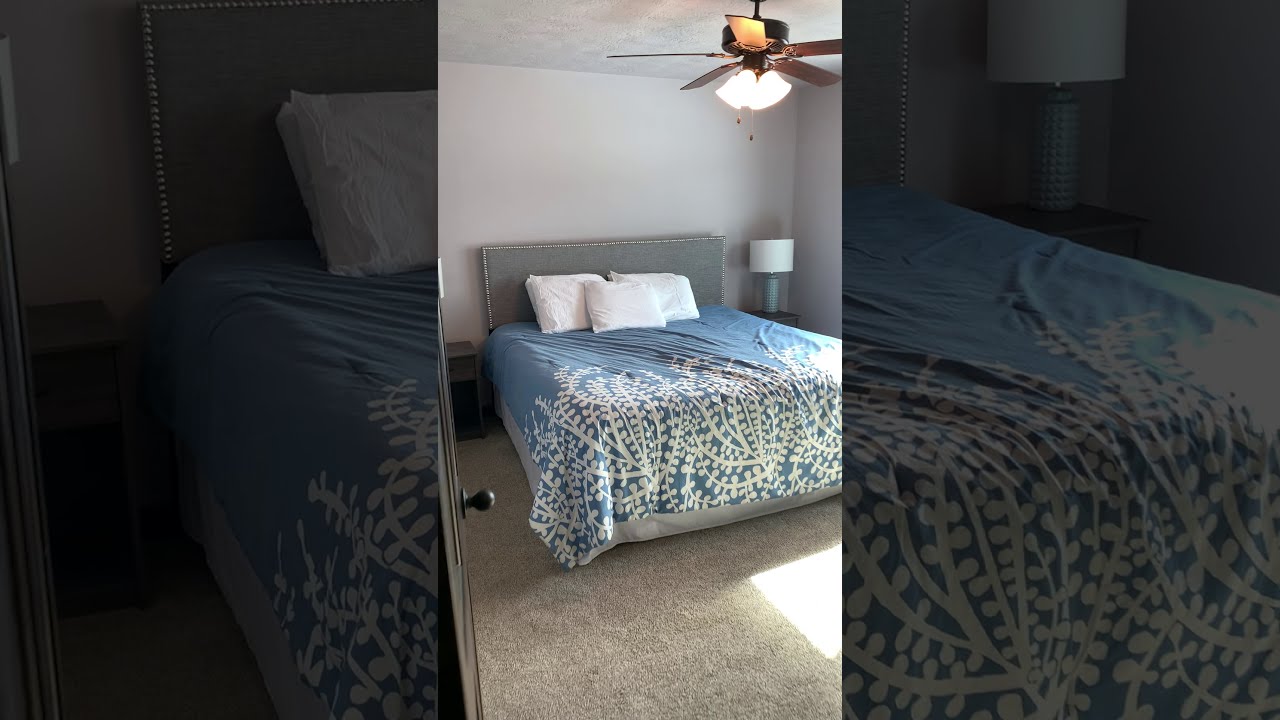The photograph captures a serene bedroom with a central focus on a queen-sized bed. The bed, positioned in the middle of the room, features a blue bedspread adorned with intricate white floral designs and three plush white pillows propped against a gray, fabric headboard with subtle silver trim. Flanking the bed are two nightstands, each hosting a light blue lamp with a white round lampshade. Above, a brown wooden ceiling fan equipped with four light bulbs illuminates the space. The room's floor is covered with a grayish, wall-to-wall carpet, and the walls and ceiling are painted white, creating a crisp and clean backdrop. The bedroom door stands open, offering a welcoming view into the cozy space. There are no people in the image, enhancing the tranquil and undisturbed atmosphere of the room.